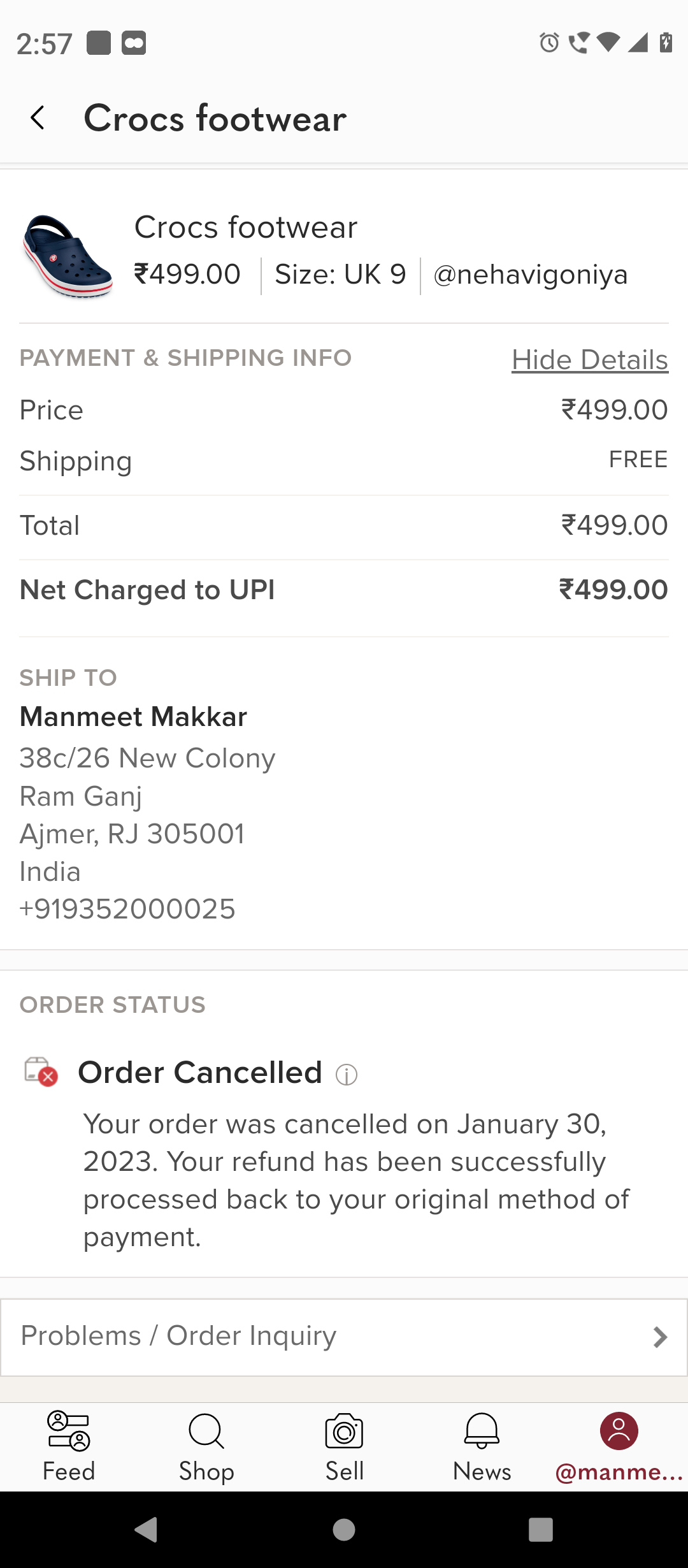This screenshot captured from a mobile phone in portrait mode presents a detailed view of a canceled footwear order. 

- **Top Section**:
  - **Top Left Corner**: An indicator showing '257'.
  - **Top Right Corner**: A fully charged battery icon.

- **Header**: 
  - A dark black bar labeled "Crocs Footwear" accompanied by a back arrow.

- **Content**:
  - Two subtle divider lines.
  - An image of blue Crocs featuring a distinctive red stripe around their white bottoms.
  - Product description: "Crocs Footwear" priced at $499. The exact currency is unspecified.
  - Size information: "Size UK 9" at the vendor "NEHAVIGONIYA".

- **Transaction Details**:
  - Price: $499.
  - Shipping: Free.
  - Total Cost: $499.
  - Payment Method: Net charge to UPI $499.
  - Shipping Address: MANMEETMAKAR, 38C-26 New Colony, Ramganj, Ajmer, RG 305001, India.
  - Phone Number: Included but obscured for privacy.
  
- **Order Status**:
  - Status: Canceled.
  - Cancellation Date: January 30th, 2023.
  - Refund: Successfully processed back to the original method of payment.
  - Action Link: Problems with the order? Inquiries can be made.

- **Navigation Bar** at the bottom includes tabs for:
  - Feed
  - Shop
  - Sell
  - News
  - User Profile (identified as "MANME")

This comprehensive breakdown provides a clear and detailed view of the information contained in the screenshot.